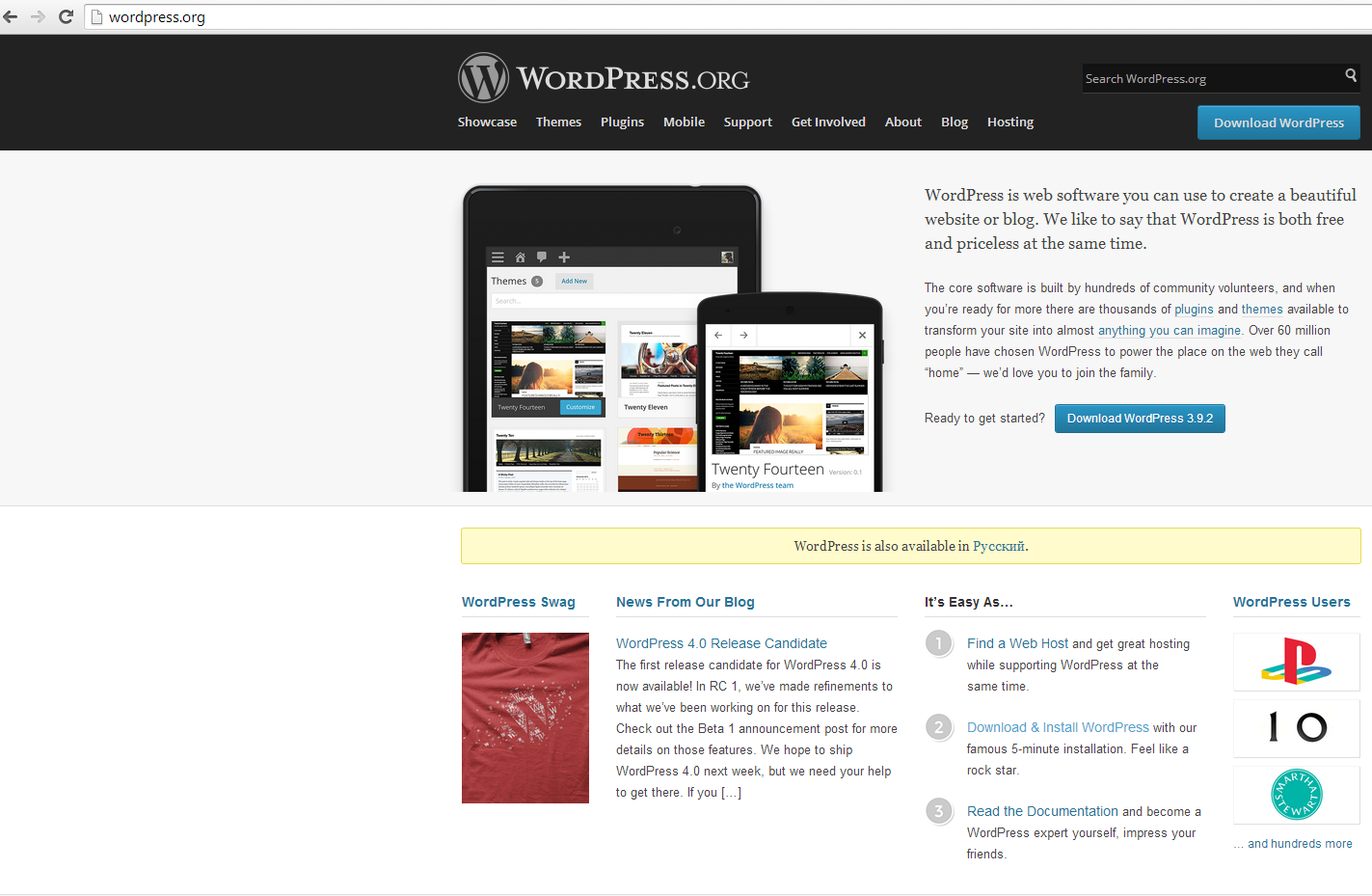The image is a screenshot of the WordPress.org homepage, showcasing various elements of the site’s interface and content. 

At the very top of the screen, you can see the browser's toolbar, complete with the back button, the forward button (which is grayed out), and the reload button depicted as a half circle with an arrow pointing clockwise. Adjacent to these is the search bar displayed within the browser interface.

The WordPress.org website interface begins with a black text search bar set against a white background. Directly below this is a dark gray banner running across the screen, featuring the text "wordpress.org" in white centered within the banner. To the left of this text is the WordPress logo, which consists of a black "W" within a light gray circle.

Below the banner, there is a navigation menu with buttons labeled "Showcase," "Themes," "Plugins," "Mobile," "Support," "Get Involved," "About," "Blog," and "Hosting." In the top right corner of the screen, there is another search bar with "search wordpress.org" in white text, set against a black background with a white magnifying glass icon at the end. Next to this search bar is a blue button with white text that reads "Download WordPress."

Moving down the page, the next section showcases an iPad or tablet alongside a mobile device, both displaying a website with a white background containing black text and photographs, which are too small to annotate specifically. Beside these devices, there is a text block that reads:

"WordPress is web software you can use to create a beautiful website or blog. We like to say that WordPress is both free and priceless at the same time. The core software is built by hundreds of community volunteers, and when you're ready for more, there are thousands of plugins and themes available to transform your site into almost anything you can imagine. Over 60 million people have chosen WordPress to power the place on the web they call home. We'd love you to join the family."

This text is rendered in black. Below it, there is another prompt saying "Ready to get started?" followed by a blue button with white text that reads "Download WordPress 3.9.2."

Further down, a light yellow banner indicates that "WordPress is also available in [a language that appears to be Hindi]." This is followed by various sections arranged horizontally:

1. **WordPress Swag**: Displays a red t-shirt bedazzled with a "W" for WordPress.
2. **News from Our Blog**: Features a segment titled "WordPress 4.0 Release Candidates," alongside a descriptive paragraph.
3. **It's Easy As...**: Lists steps in blue text: 
   - "1. Find a web host"
   - "2. Download and install WordPress"
   - "3. Read the documentation"
4. **WordPress Users**: Features logos including the PlayStation logo, a logo that reads "IO" or "10," and the Martha Stewart logo inside a light green circle. This section concludes with the text "...and hundreds more" in blue.

Overall, the image illustrates a detailed and highly structured layout of the WordPress.org homepage, providing a comprehensive overview of its various functions and features.